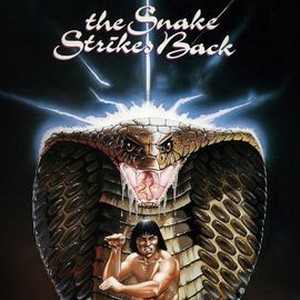Set against a black background, this striking graphic appears to be a movie poster titled "The Snake Strikes Back," written in white cursive text at the top. Dominating the center of the image is a colossal hooded cobra with brown scales, its menacing eyes piercing towards the viewer. The cobra's mouth is wide open, revealing sharp fangs and dripping venom, while jagged streaks of white lightning illuminate its head, adding an electrifying aura.

Beneath the cobra, a shirtless man with long, dark hair stands ready in a martial arts pose. His right arm is bent at the elbow, raising his fist towards his face, while his left arm extends outward with his palm facing down, prepared to block incoming attacks. The disproportionate size of the snake compared to the man enhances the dramatic and overpowering presence of the cobra, creating a dynamic and intense visual impact.